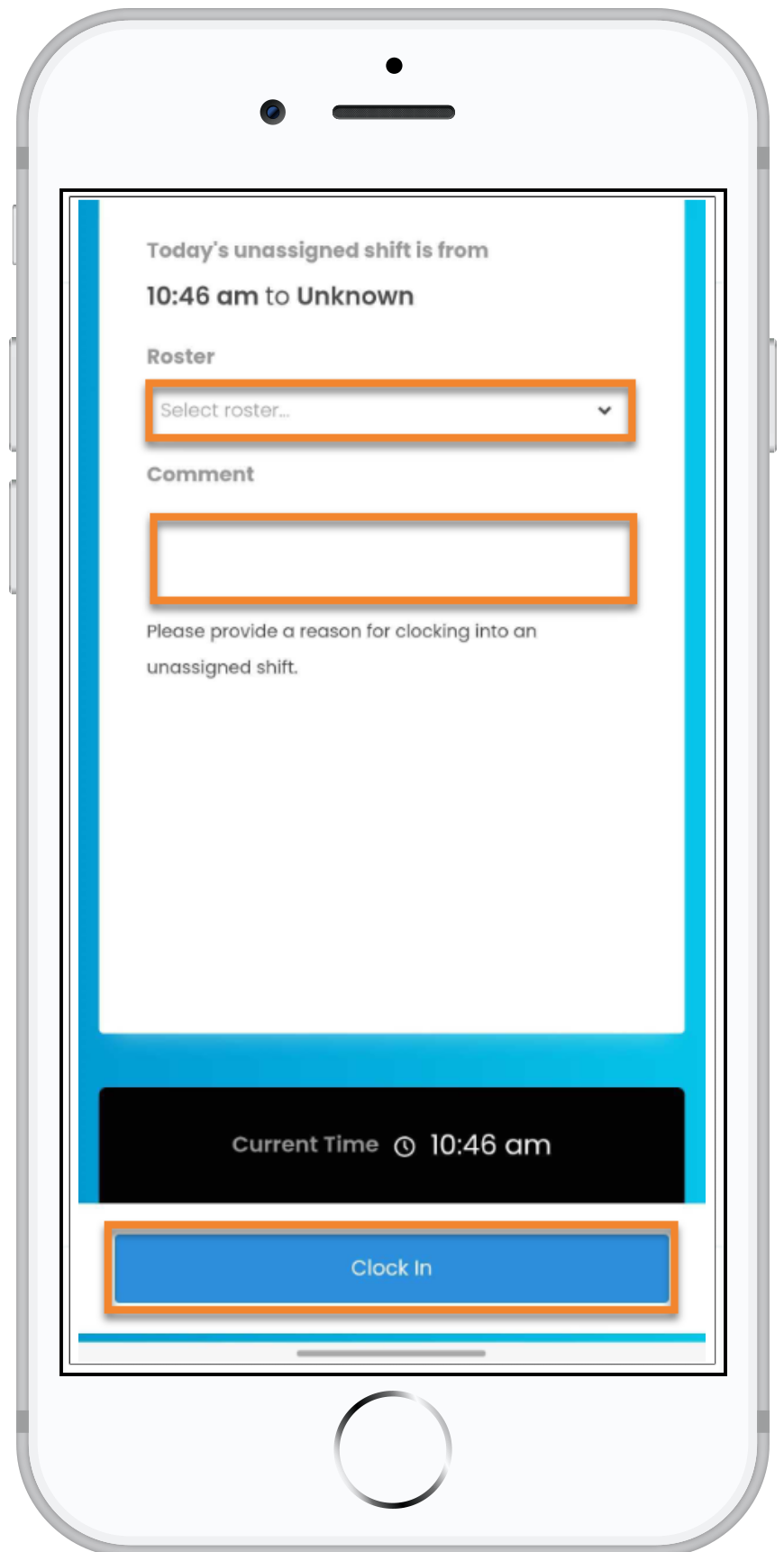**Image Description:**

The image delineates an outlined smartphone interface. The smartphone's outline is depicted with a gray line on a white background. Centered in this outline, there is a small black dot, representing a feature of the phone, perhaps a camera lens. To the right of this dot, a larger black dot is situated, accompanied by a black line beside it, and another black line positioned underneath it.

Midway down the interface, there are two blue bars on either side. Displayed in black font, the text reads: "Today's unassigned shift is from," followed by the time "10:46 a.m." and the word "Unknown." Below this, another section labeled "Roster" is shown, characterized by an orange square with a white interior and gray font that states "Select roster." Adjacent to this section is a downward-facing black arrow icon.

Further down, the word "Comment" is written, succeeded by another orange square with a white interior. Beneath this, text in gray font prompts: "Please provide a reason for clocking into an unassigned shift."

Toward the bottom of the screen, there is a gray box followed by a blue box containing a smaller black box. In white font within the blue box, it reads "Current Time," alongside a white clock icon displaying "10:46 a.m."

The image also includes an orange-box outline, below which a gray background and blue interior are featured, with white font over it stating "Clock In." A blue line separates it from a gray line beneath.

The outermost regions of the outline consist of a finished black and gray border. Toward the left side, two gray buttons are placed vertically, and along the right side, another singular gray button is positioned, mirroring the physical buttons typically found on a smartphone.